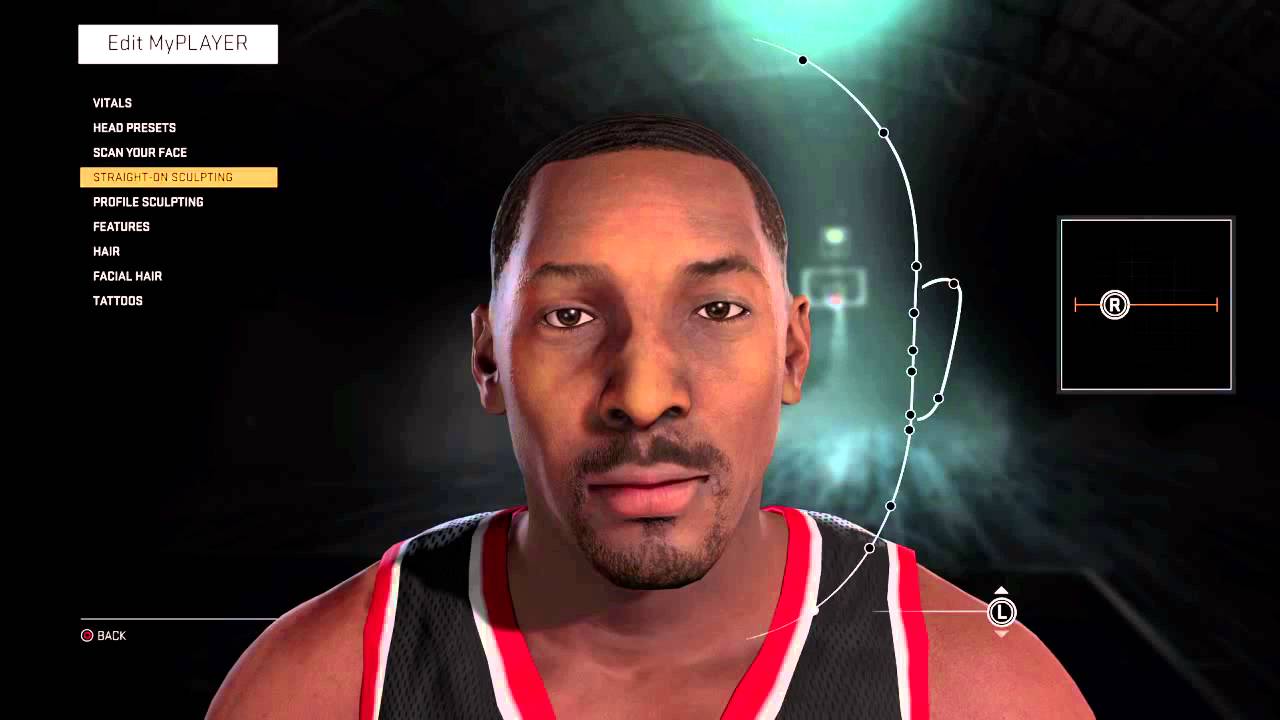The image appears to be a screenshot from a video game where players can create and customize their own basketball player. At the top of the interface, there is a grey box with the text "Edit My Player" in black letters. Below this title, several customization options are listed in white text: "Vitals," "Head Presets," "Scan Your Face," "Straight When Sculpting," "Profile Sculpting," "Features," "Hair," "Facial Hair," and "Tattoos." The option "Straight When Sculpting" is currently selected, highlighted with a yellow box.

The background is predominantly black, drawing focus to the center where there is a green-colored light and an indistinct image behind it. On the right side of the screen, there is a white box featuring a brown bar and a white circle with the letter "R" inside it. 

In the middle of the interface is an image of the customized basketball player. The player has dark skin, dark eyes, and very short dark hair. The athlete is wearing a red, black, and white striped basketball jersey. Below the image of the player’s face, there is a white line with a circle containing a white "L" and up and down arrows, possibly indicating navigation controls. To the left of the player, there is another white line with the word "Back" and a red circle, suggesting an option to return to the previous menu.